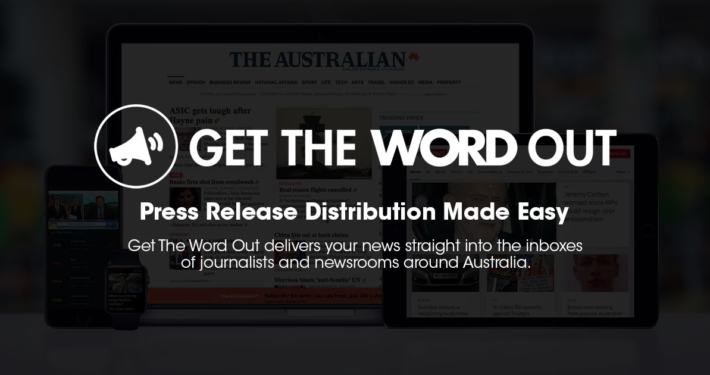The image showcases a website with a sleek black background, juxtaposed against a display of various technological devices, including a computer monitor, an iPad, a smartphone, and a smaller device that appears to be a smartwatch. The computer screen prominently features the website "The Australian," indicating its focus on news distribution in Australia. In the foreground, the website's header reads, "Get the word out," accompanied by a graphic of a megaphone emitting lines to simulate speech. Below the header, the text promotes the service by stating, "Press release distribution made easy. Get the word out delivers your news straight into the inboxes of journalists and newsrooms around Australia." The devices are placed on a pristine white surface, and the background includes window panels, suggesting a professional and modern setting.